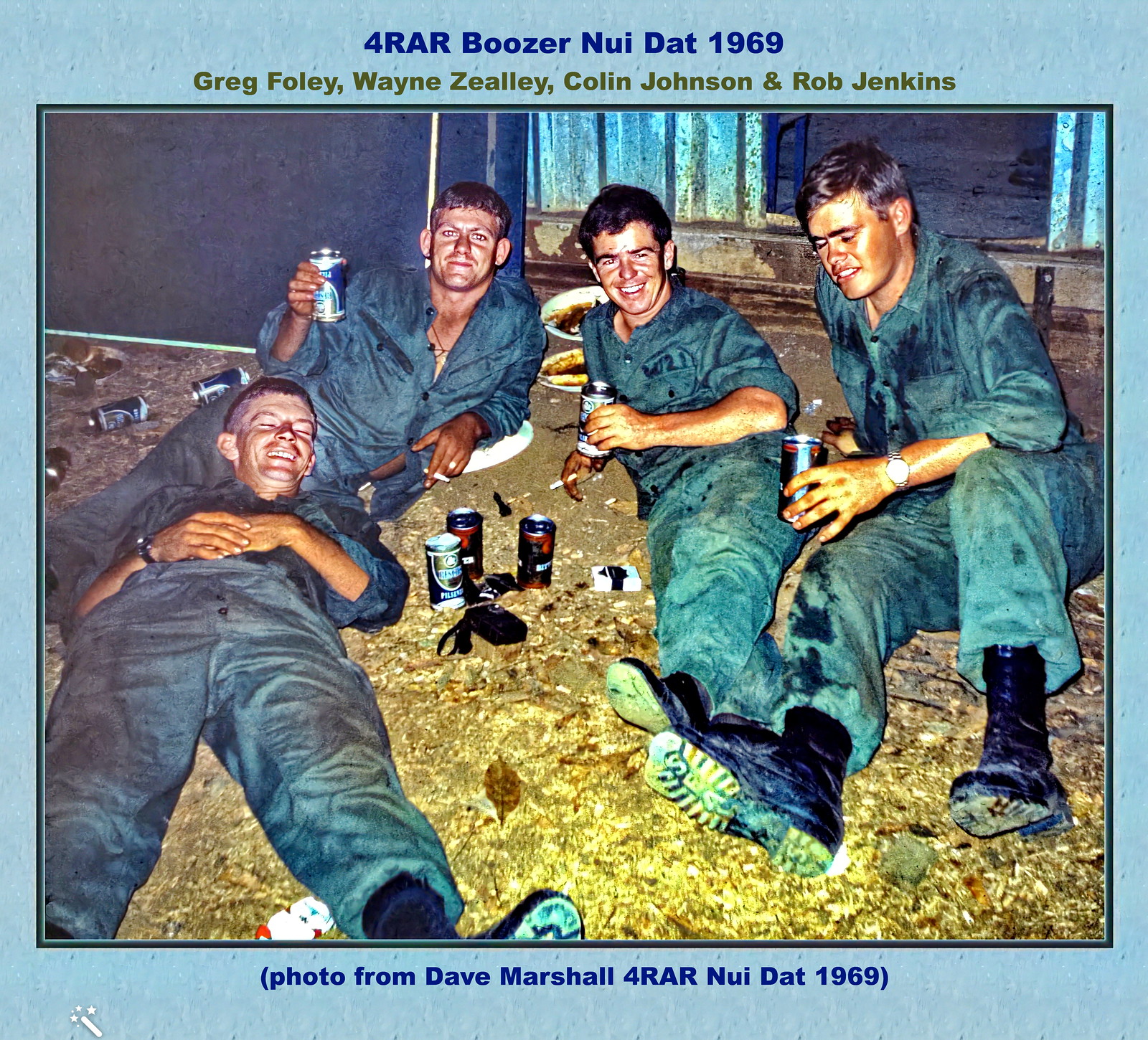This is an aged color photograph from 1969 depicting four soldiers during the Vietnam War, specifically labeled as For 4RAR Boozer Nui Dat 1969. Encased by a blue-bordered frame, the photograph features Greg Foley, Wayne Zeeley, Colin Johnson, and Rob Jenkins, all identified in green text below the image. Lying on a dirt and straw-covered ground, the soldiers are dressed in worn green fatigues and black boots, surrounded by cans of beer, with three of them holding a beer each, and some plates of food seen in the background. They have relaxed postures and are smiling at the camera, suggesting a moment of camaraderie. The bottom of the frame, in dark blue text, credits the photo to Dave Marshall, indicating his presence in this informal gathering.